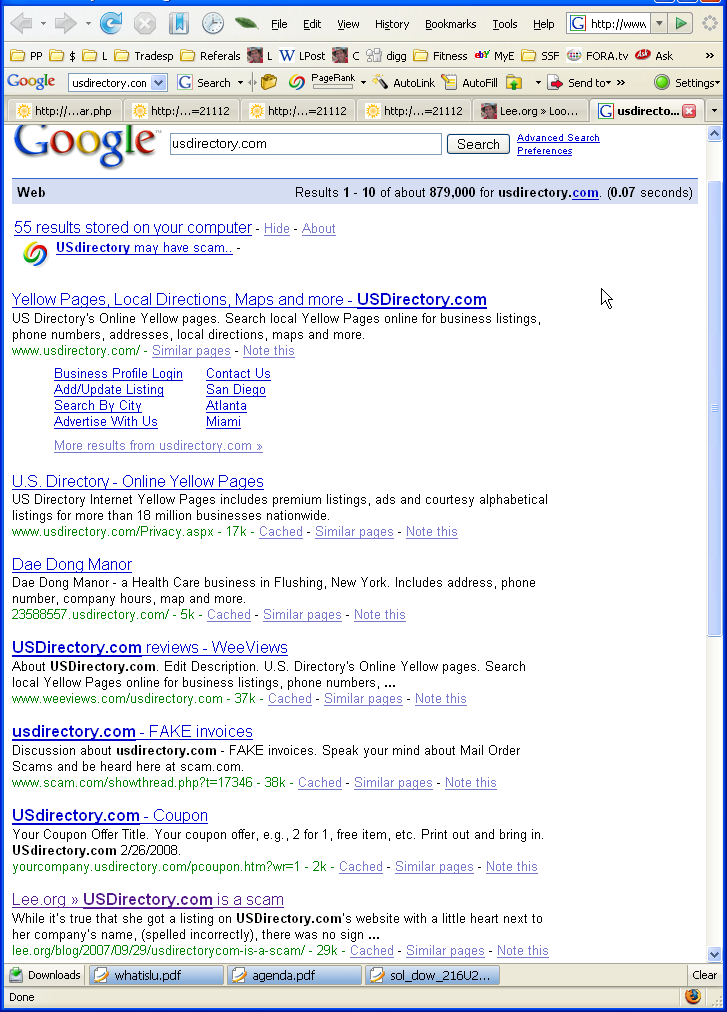A browser window displaying multiple bookmarked items and an active Google search is open on a desktop screen. The browser's search bar contains the phrase "usdirectory.com" and the displayed search results numbered one to ten show approximately 879,000 results in 0.07 seconds. The first result, highlighted and slightly different from the others, mentions "55 results stored on your computer" and addresses potential scam concerns with "usdirectory." The subsequent links lead to various related pages, including "Yellow Pages, Local Directions, Maps, and More" on usdirectory.com, and "usdirectory Online Yellow Pages." Additional links direct to "DAE DONG Manor," "usdirectory.com reviews" on "WEEVIEWS," and one on "fake invoices" with "FAKE" emphasized in capital letters. There's also a link for "usdirectory.com coupons," and the bottom-most result, from "lee.org," marks "usdirectory.com as a scam," distinguished by its purple color, signifying a previously visited site. Additionally, six tabs are open in the browser, alluding to a busy session of web navigation and research.